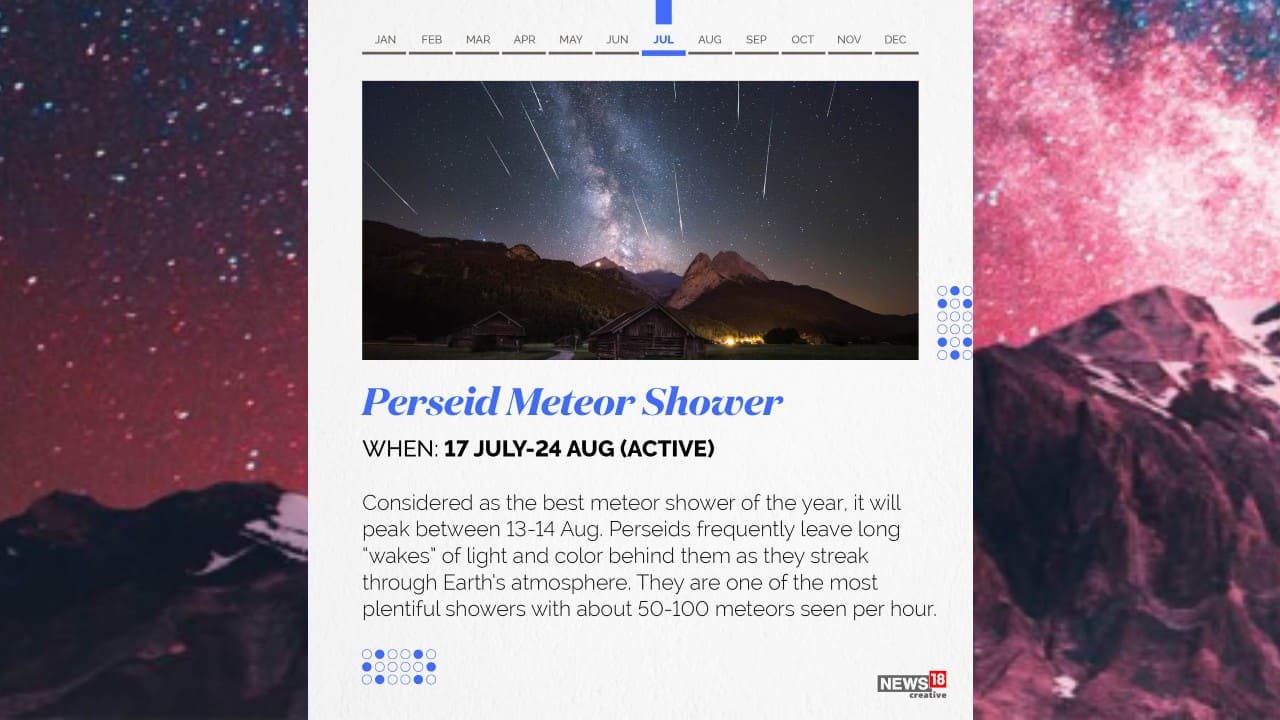This image is a screenshot of a computer screen, featuring a detailed visual representation of the Perseid Meteor Shower. The background displays a tranquil mountain range with scattered snow-capped peaks, set against a mesmerizing night sky filled with numerous stars. On the right side of the image, a densely packed cluster of stars suggests the presence of the Milky Way, enhancing the celestial display. The entire scene has a reddish tint, adding a warm, otherworldly quality to the visual.

Centrally overlaid on this background is a white text box providing detailed information about the Perseid Meteor Shower. The text states, "Perseid Meteor Shower: Active from July 17th through August 24th." It denotes that this meteor shower is considered the best of the year, with its peak expected between August 13th and 14th. The box further elaborates that the Perseids are known for leaving long trails of light and color as they blaze through Earth's atmosphere, with an impressive frequency of 50 to 100 meteors per hour. 

Above the textual content within this central box, there is an image depicting mountains beneath a sky streaked with meteor trails, visualizing what viewers might expect during the meteor shower. At the top of the box, a timeline spans from January to December, with "July" prominently highlighted, marking the observation period for this astronomical event. This well-structured and informative screenshot serves as a compelling visual guide to the upcoming Perseid Meteor Shower.